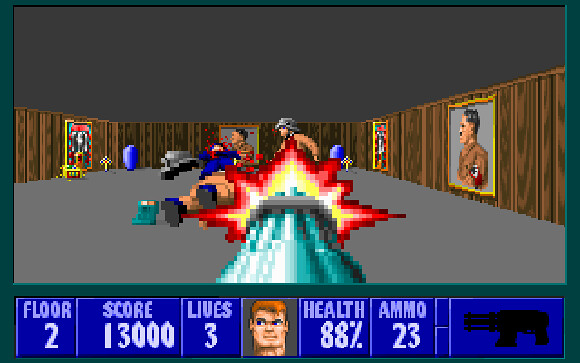This screenshot appears to be from an old-school first-person shooter video game. The setting is a portrait gallery within a museum, identifiable by the wood-paneled walls adorned with various paintings. The scene captures an intense moment: a large bomb blast is visible, and several people are lying on the ground, implying recent conflict or action. In the lower-left corner, the interface shows the player is on "Floor 2" with a score of approximately 13,000 points and three lives remaining. The player character, a white male with reddish hair and a square jaw, is displayed along with key status indicators: 88% health and 23 rounds of ammunition. The player's weapon, a black automatic gun, is depicted in the bottom-right corner of the screen.